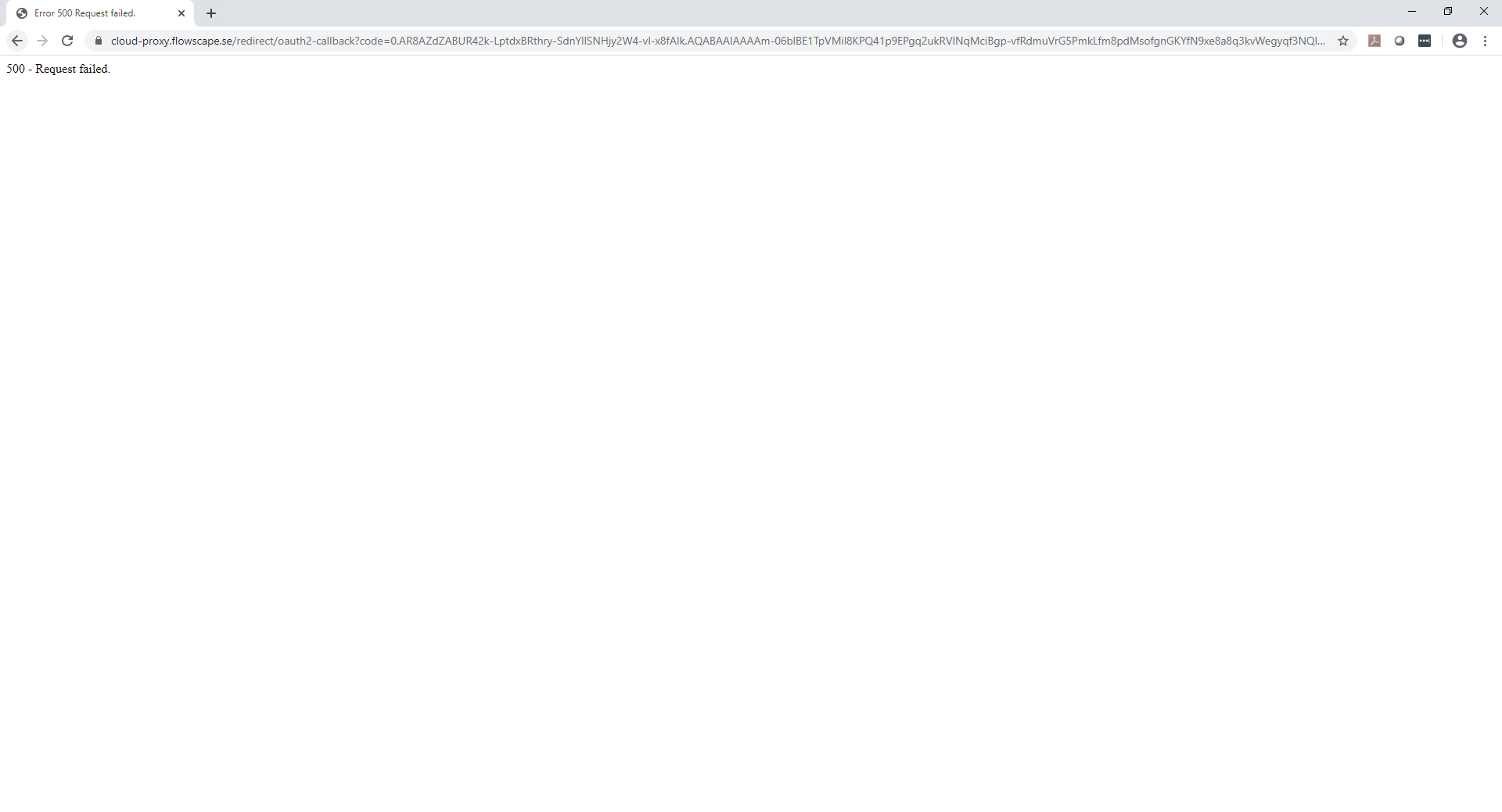The image depicts a screenshot of a computer search page with an error message prominently displayed. At the top, the header includes some text and a hyperlink, though the link is in a very small font and is nearly illegible. Dominating the screen is an error message stating "Error 500: Failed Cloud Proxy Flowscape Redirect," indicating that the search request was unsuccessful. The message further elaborates with "500: Requests Failed." Apart from the error message, the rest of the page appears blank, highlighting the disruption in the search process.